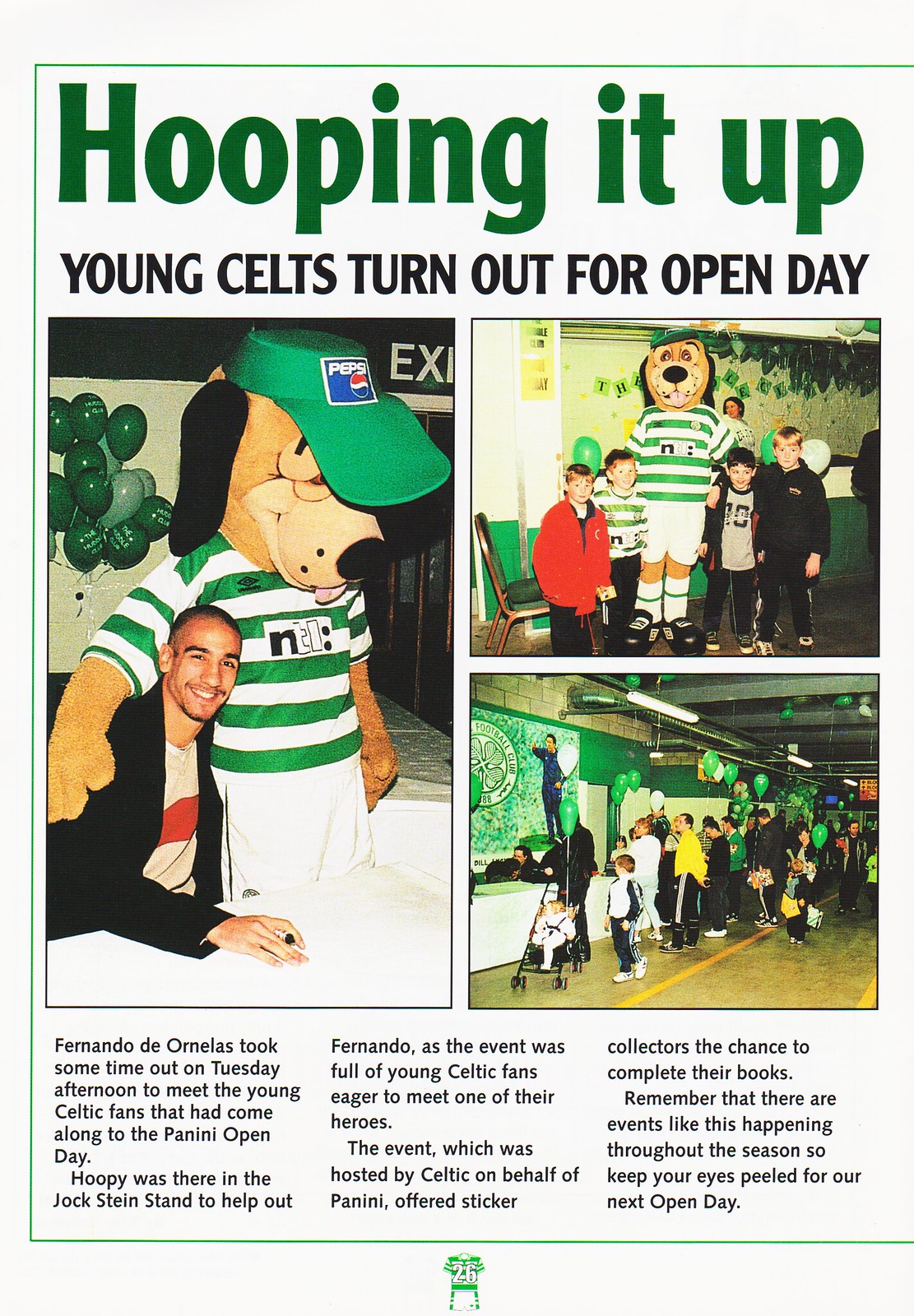The image appears to be a magazine page with a white background, bordered on three sides by a green outline, and features the headline "HOOPING IT UP" in dark green ink. Below this headline, in capital black letters, is the subheading "YOUNG CELTS TURN OUT FOR OPEN DAY." The page contains three photographs and descriptive text divided into three columns beneath them.

The first photograph is vertically oriented and depicts a man with dark hair seated and hugging a dog mascot. This mascot, characterized by its floppy ears, wears a green visor adorned with a Pepsi logo and a green and white striped shirt paired with white pants. In the background, green balloons are visible.

The second, smaller horizontal photograph on the top right shows the same dog mascot surrounded by four children in what appears to be a classroom setting. The mascot affectionately huddles with the children, enhancing the celebratory atmosphere.

The third photograph at the bottom displays a scene of various people lined up, holding green umbrellas and possibly receiving balloons at a table. This image reflects the communal and festive nature of the event.

Lastly, the accompanying text articulates that Fernando de Ornez participated in the event on Tuesday afternoon, taking time to meet the young Celtic fans during the Panini Open Day. The dog mascot, Hoopy, was present in the Jock Stein stand to support Fernando, as the event was bustling with enthusiastic young fans eager to greet their sports hero. The event, arranged by Celtic in collaboration with Panini, provided an opportunity for sticker collectors to complete their collections. The text also encourages fans to stay informed about upcoming open day events throughout the season.